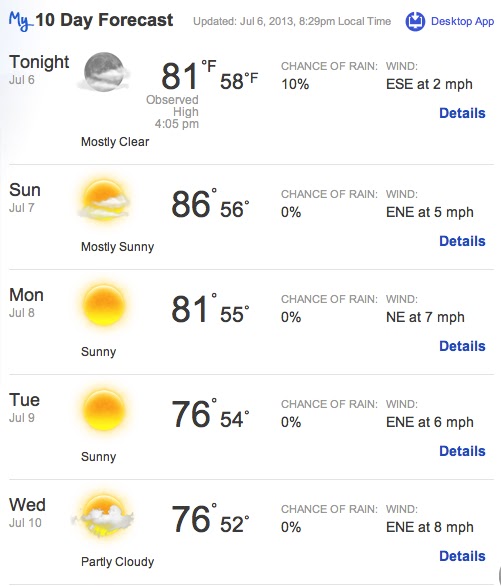The image depicts a 10-day weather forecast starting from the top left corner, which shows the date "May" and a title reading "10 Day Forecast." The forecast was updated on July 6, 2013, at 8:29 p.m. local time.

To the top left, a blue circle is present, labeled as "Tessaga."

For July 6, the center section shows:
- Mostly clear weather.
- Observed temperatures: High of 80°F at 4:05 p.m., Low of 60°F.
- Chance of rain: 2%.
- Wind: East-Southeast at 2 mph.

For July 7:
- Mostly sunny.
- Temperatures: High of 86°F, Low of 56°F.
- Chance of rain: 2%.
- Wind: East-Northeast at 5 mph.

For July 8:
- Strongly sunny.
- Temperatures: High of 81°F, Low of 55°F.
- Chance of rain: 0%.
- Wind: East-Northeast at 7 mph.

For July 9:
- Sunny.
- Temperatures: High of 76°F, Low of 54°F.
- Chance of rain: 0%.
- Wind: East-Northeast at 6 mph.

For July 10:
- Partly cloudy.
- Temperatures: High of 76°F, Low of 52°F.
- Chance of rain: 0%.
- Wind: East-Northeast at 8 mph.

The background of the image is white, and there are dividing lines between each day's forecast.